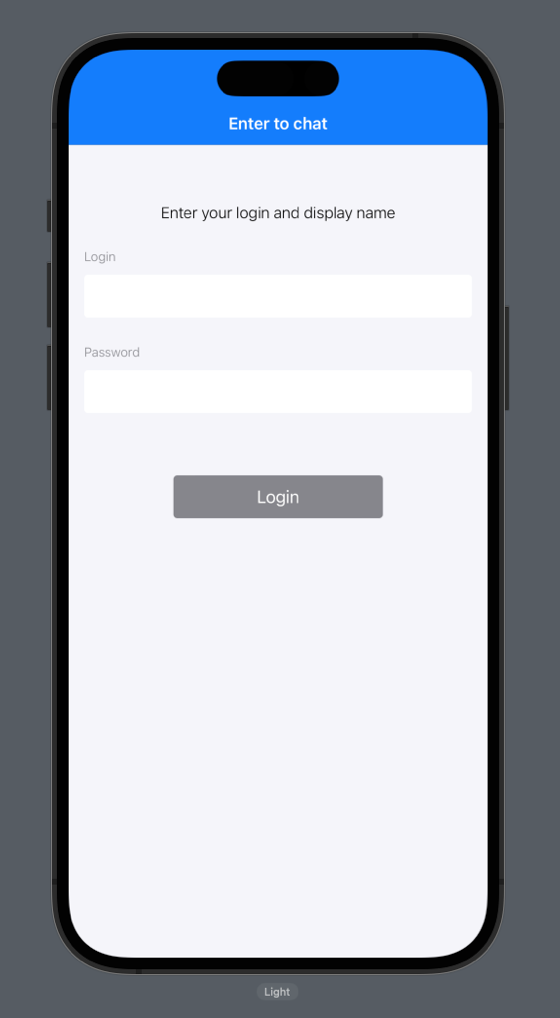This image is a stylized screenshot of a mobile device's login screen. The mobile device itself has a sleek, black frame, clearly visible against the surrounding dark, light gray background. Within the device's screen, the top section is dominated by a horizontal blue banner. In the center of this banner, it indicates with white text: "Enter to chat."

Below this blue section, the main part of the screen features a light gray background with instructions in the middle: "Enter your login and display name." Directly underneath this prompt are two empty text fields, rectangular in shape and white in color. The upper text field is labeled "Login" in light gray text, while the one beneath it is labeled "Password" in the same style.

A significant portion of the lower screen is occupied by a dark gray button with the word "Login" centered in white letters. At the top of the screen, there are some navigation buttons—one situated in the top left corner and another in the top right, although their specific functions are not detailed.

Outside the confines of the phone screen, on the encompassing background, there is a noticeable light gray oval positioned at the bottom center with the word "Light" inscribed in white letters.

This composition creates a clear and user-friendly visual emphasizing the login interface of the mobile application.